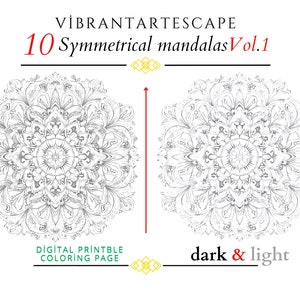The image is a promotional digital printable coloring page from a coloring book. At the top, the text in black reads "Vibrant Artscape," followed by the number "10" in red, then "Symmetrical Mandalas" in black, and "Volume 1" in red. Below this, there are two intricate mandala patterns, one on the left and one on the right, both created with multiple layers of petals arranged in a floral design. These mandalas are separated by a vertical red line. At the bottom of the image, in green text on the left, it states "Digital Printable Coloring Page," and on the right, it mentions "Dark and Light." The mandalas on this page can be colored in any colors the user chooses.